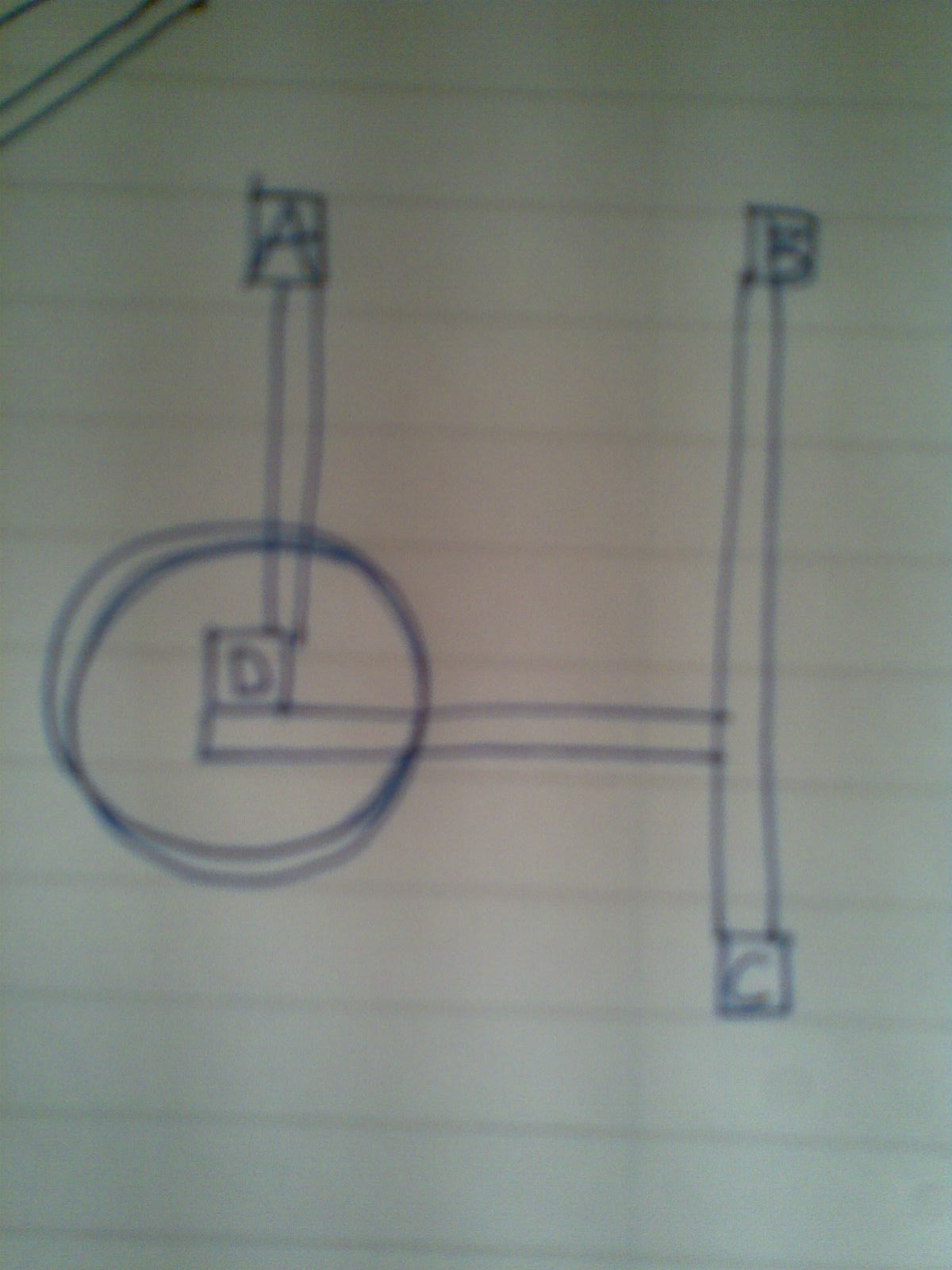This photograph features a close-up view with a vertical orientation of a piece of white-lined paper. The paper contains a simple drawing executed with a blue pen or marker. In the lower left-hand corner of the image, there are two overlapping circles resembling wheels. Extending from these circles are three distinct bars: one vertical bar extending upward from the center of the wheels, another horizontal bar extending to the right, and a third vertical bar positioned perpendicular to the horizontal bar. Together, these bars form a shape that resembles an open-topped number four. Additionally, there are some diagonal lines situated in the upper left-hand corner of the paper, adding extra detail to the otherwise minimalist composition.